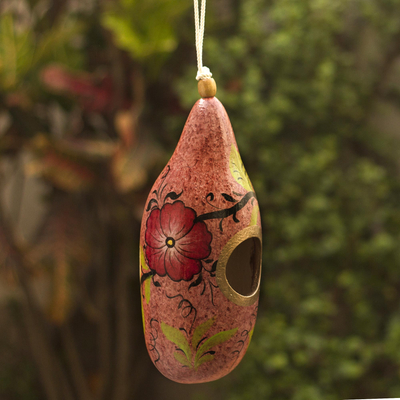A photograph captures an intricately designed bird feeder crafted from a dried husk resembling a pomegranate. It hangs suspended in the air by a white string attached through a small yellow section at the top. The husk boasts a captivating mix of reddish and dark red hues, enhanced with hand-painted details. Prominently featured is a vivid red flower with a yellow, orange center, surrounded by black embroidered accents. Intertwined vines and leaves, in shades of black and green, extend from the top right to the bottom left of the feeder, adding a dynamic texture to its surface. There's a noticeable hole on the right side, rimmed with a golden ring, revealing a grayish interior. The feeder's picturesque setting is lit by sunlight, though the surrounding vegetation and what appears to be a secondary birdhouse remain softly blurred in the background, hinting at a lush, serene outdoor environment.